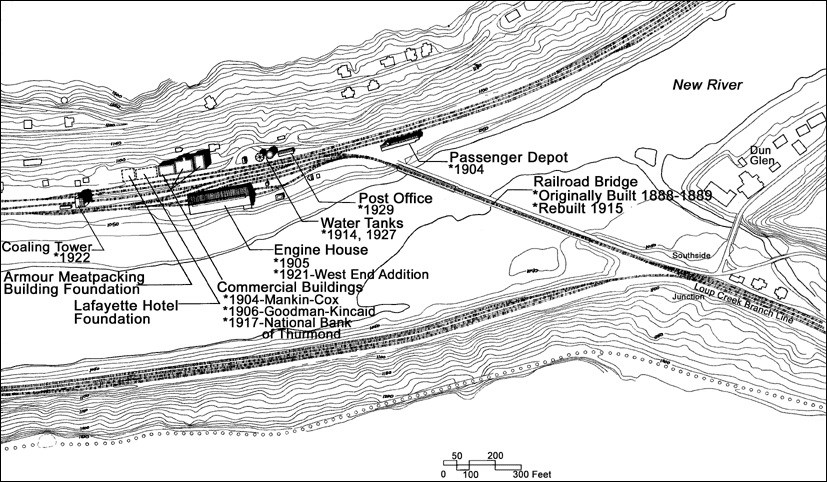The image is a detailed, black and white, hand-drawn map depicting a historical town layout beside New River, near Dunn Glen. The map is marked by numerous squiggly lines that likely represent rivers or terrains and includes various labeled locations, each with specific dates, indicating their historical significance. Prominent locations include the Railroad Bridge built between 1886-1889 and rebuilt in 1915, the Passenger Depot from 1904, the Post Office from 1929, and Water Tanks from 1914 and 1927. The map also highlights the Engine House (1905, with a 1921 West End Addition), several commercial buildings including the Mankin-Cox Building (1906), the Goodman-Kincaid Building (1917), and the National Bank of Thumbolt. Other notable structures are the Coaling Tower from 1922, the Armor Meatpacking Building Foundation, and the Lafayette Hotel Foundation. A measurement indication is faintly visible at the bottom of the map, adding to the historical depth and context of this town layout.